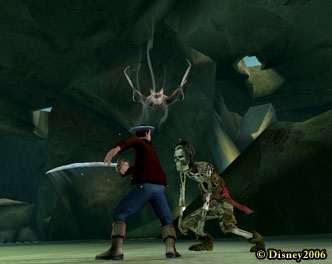The image, captioned "Disney 2006" in yellow text at the lower right corner, depicts a dramatic scene set in a cave with a predominantly green background and greenish-brown rocks. The focal point is a man dressed in blue jeans, brown boots, and a dark plum-colored long-sleeved shirt. Wearing a hat, he is poised for action with a sword held in his right arm, which is pulled back, preparing to strike. His side profile and determined posture suggest readiness for combat. Facing him is a zombie-like creature, characterized by its decayed appearance, partial skeleton, and long hair. It is hunched over with ragged clothes hanging from its frame and dark, hollow eyes. Above them hovers a large, white-faced bat-like creature with extended arms, seemingly ready to join the fray. The cave setting is dimly lit with patches of blue sky visible through holes in the rocky structure, giving it a sense of depth and foreboding atmosphere. The floor of the cave is a lighter green, emphasizing the eerie environment where the confrontation unfolds.